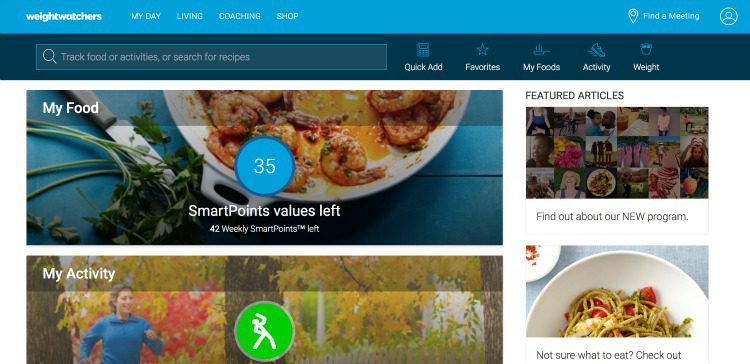This image showcases the homepage of the Weight Watchers website. At the top, a light blue navigation bar stretches across the width of the screen. On its left side, the "Weight Watchers" logo is prominently displayed. To the right of the logo, there are four menu options: "My Day," "Living," "Coaching," and "Shop." 

Beneath this, a darker blue navigation bar features a search function that reads "Track food or activities or search for recipes." This search bar is flanked on the right by several quick-access links: "Quick Add," "Favorites," "My Foods," "Activity," and "Weight."

The main content area below the navigation bars is titled "My Food." It features a visually appealing image of a plate with shrimp, positioned slightly to the left. Dominating the center of this section is a prominent blue circle displaying the number "35." Directly underneath this circle, the text "SmartPoints" is displayed, followed by "Values Left." Below that, the text "42 Weekly SmartPoints Left" is present, indicating remaining points for the week.